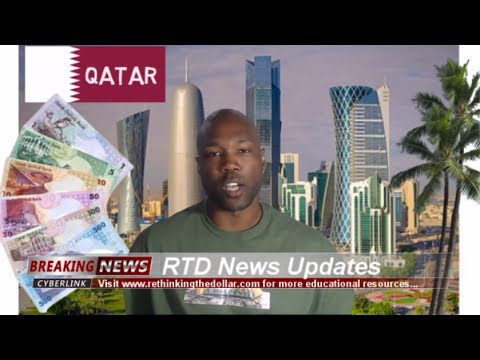The image depicts an African gentleman, bald and dressed in a dark green t-shirt, standing amidst a breaking news broadcast set against the backdrop of the distinctive skyline of Qatar. The background features an array of unique skyscrapers: one cylindrical and silver, another shiny with pointed edges, and a third that curves to one side. To the man's left, foreign currency in pink, green, and red shades is fanned out prominently, while two palm trees stand to his right. A burgundy overlay at the upper left corner bears the word "Qatar" in white letters. Superimposed across the lower part of the scene is a transparent banner with the text: "Breaking News, RTD News Update, Cyberlink. Visit www.rethinkingthedollar.com for more educational resources," written in a mix of red, white, and black fonts. This composition suggests a TV news screenshot, with the man appearing mid-speech, adding urgency and immediacy to the scene.